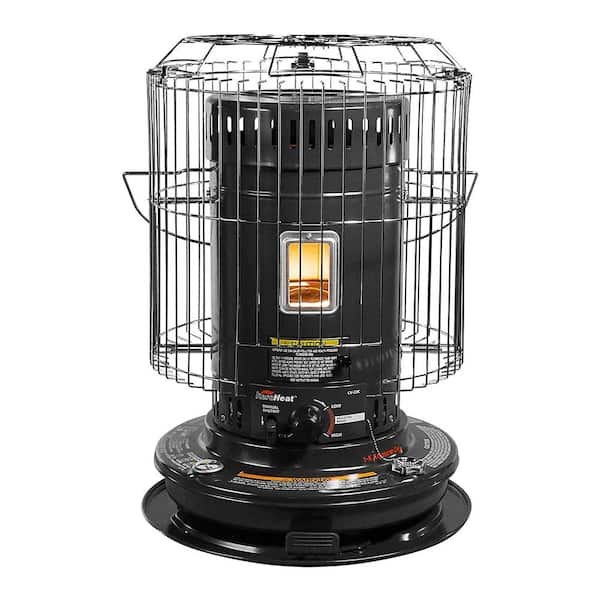The image displays a detailed color photograph of a black kerosene heater on a white background. The heater features a cylindrical core with a prominent black base that supports the structure and prevents tipping. At the heart of the unit is a small window framed in metallic silver, revealing the inner flame with yellow and orange hues. Above the black base, the cylinder showcases yellow and white lettering, likely containing operational instructions and caution warnings. A notable black round dial, positioned below the text, allows for adjusting the temperature settings, indicating levels from low to high.

Encasing the entire heater is a chrome-colored protective cage, designed to prevent accidental burns by shielding the user from direct contact with the hot surfaces. This cage extends from the top to a few inches above the base, providing both safety and stability. The overall design is reminiscent of protective structures like bird cages or mailboxes found in the United Kingdom. The heater is adorned with multiple warning labels and cautionary notes for safe operation.